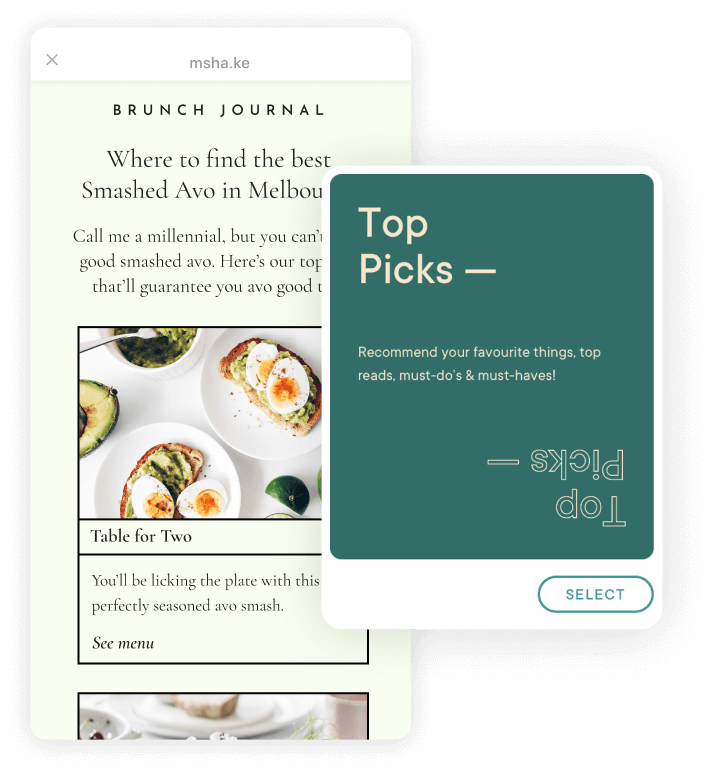The image consists of two vertically-oriented mobile screen snapshots, with one slightly superimposed over the other. The smaller image, positioned on top, displays a UI section titled "Top Picks," featuring categories such as "Recommended," "Recommend Your Favorite Things," "Top Reads," and "Must Do's and Must Haves," along with a clickable "Select" button.

In the background, the larger, partially obscured image showcases a webpage from msha.ke, identified as "Brunch Journal." The visible heading reads, "Where to Find the Best Smashed Avo in Melbourne," followed by a partially cut-off sentence beginning with "Call me a millennial, but..." This background image appears to be part of a food app, prominently featuring a photograph of an elegantly arranged plate. The dish includes deviled eggs on toast and avocado, set against a beige backdrop, presenting a visually appealing food setup.